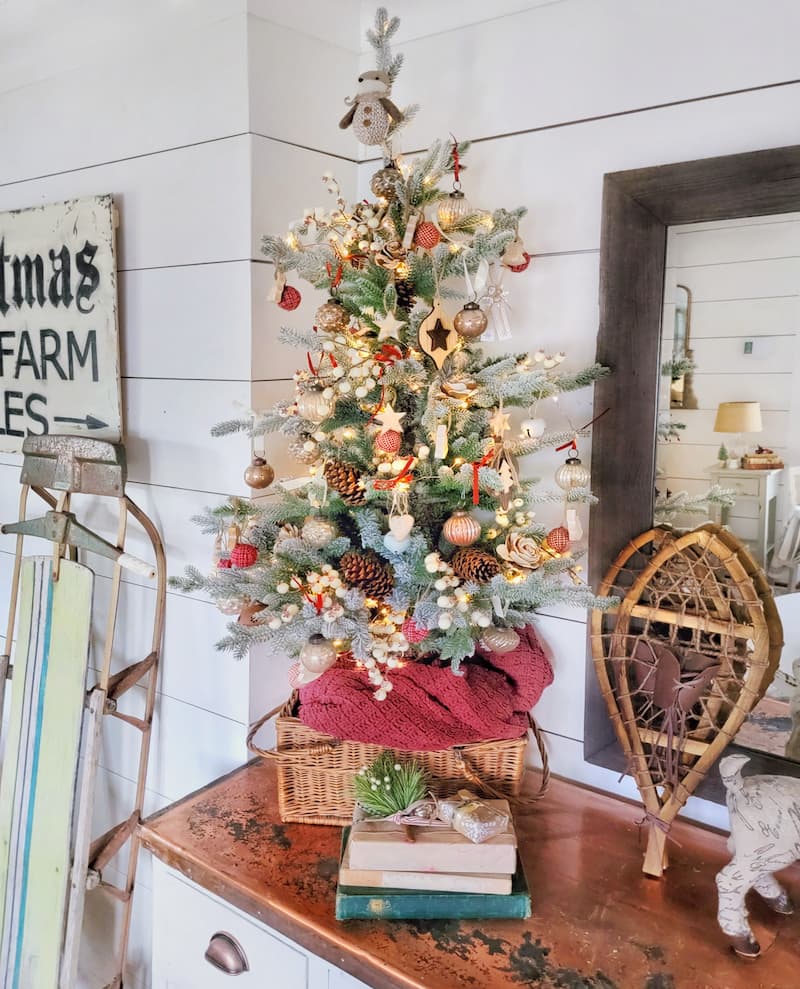The image showcases a charming country-style indoor holiday vignette centered around an antique dresser, now repurposed with a beautifully intricate slab of wood as its top. Atop the dresser sits a small, heavily decorated Christmas tree, about two to three feet tall, nestled in a basket. The tree is adorned with an array of ornaments, including natural elements like pine cone and acorn ornaments, popcorn garlands, old-fashioned glass balls, artificial roses, and a soft, plushy figure topping the tree. Surrounding the tree is a collection of books and possibly a wrapped present or two. 

To the left of the dresser, propped against a white wooden wall, is an old-fashioned runner sled, and above it is a partially visible sign reading "Christmas... farm" and "trees," with an arrow pointing right, suggesting a Christmas tree farm. Resting below a rustic wooden-framed mirror are toy-sized snowshoes. The mirror captures the reflection of a side table and lamp, adding depth to the cozy, farmhouse-style ambiance. The scene is completed by the partially visible rear legs of a goat or horse statue, adding a subtle touch of whimsy to the rustic holiday decor.